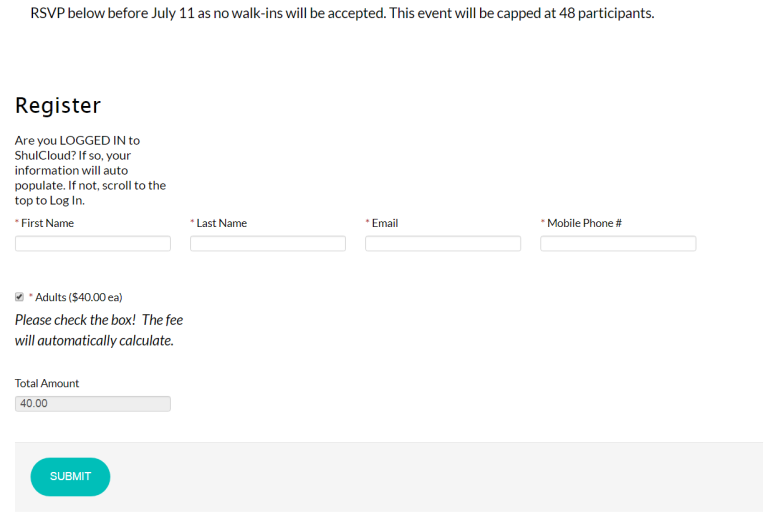The screenshot depicts a website's event registration page, providing a structured layout for securing a spot at an upcoming event. At the top of the page, a prominent notice states, "RSVP by July 11th as no walk-ins will be accepted," emphasizing the importance of early registration. The event is limited to 48 participants.

Below this notice, the page title, "Register," is displayed, accompanied by a query, "Are you logged into Show Cloud?" indicating an affiliation with the Show Cloud platform and implying that login might be required for registration.

The main section includes four mandatory fields, each marked with a red asterisk: First Name, Last Name, Email, and Mobile Phone Number. These fields ensure that the registrant's basic contact information is collected. Additionally, there's a checkbox labeled "Adults, $40 each," which is already checked, bringing the total amount due to $40.

At the bottom of the registration form is a green "Submit" button, guiding users to finalize their registration. Although the image provides no further information about the event's nature—whether it's a movie screening, party, sporting event, or otherwise—it clearly outlines the registration process up to the point of payment confirmation, in adherence to the rules that no walk-ins will be admitted and participation is capped at 48 individuals.